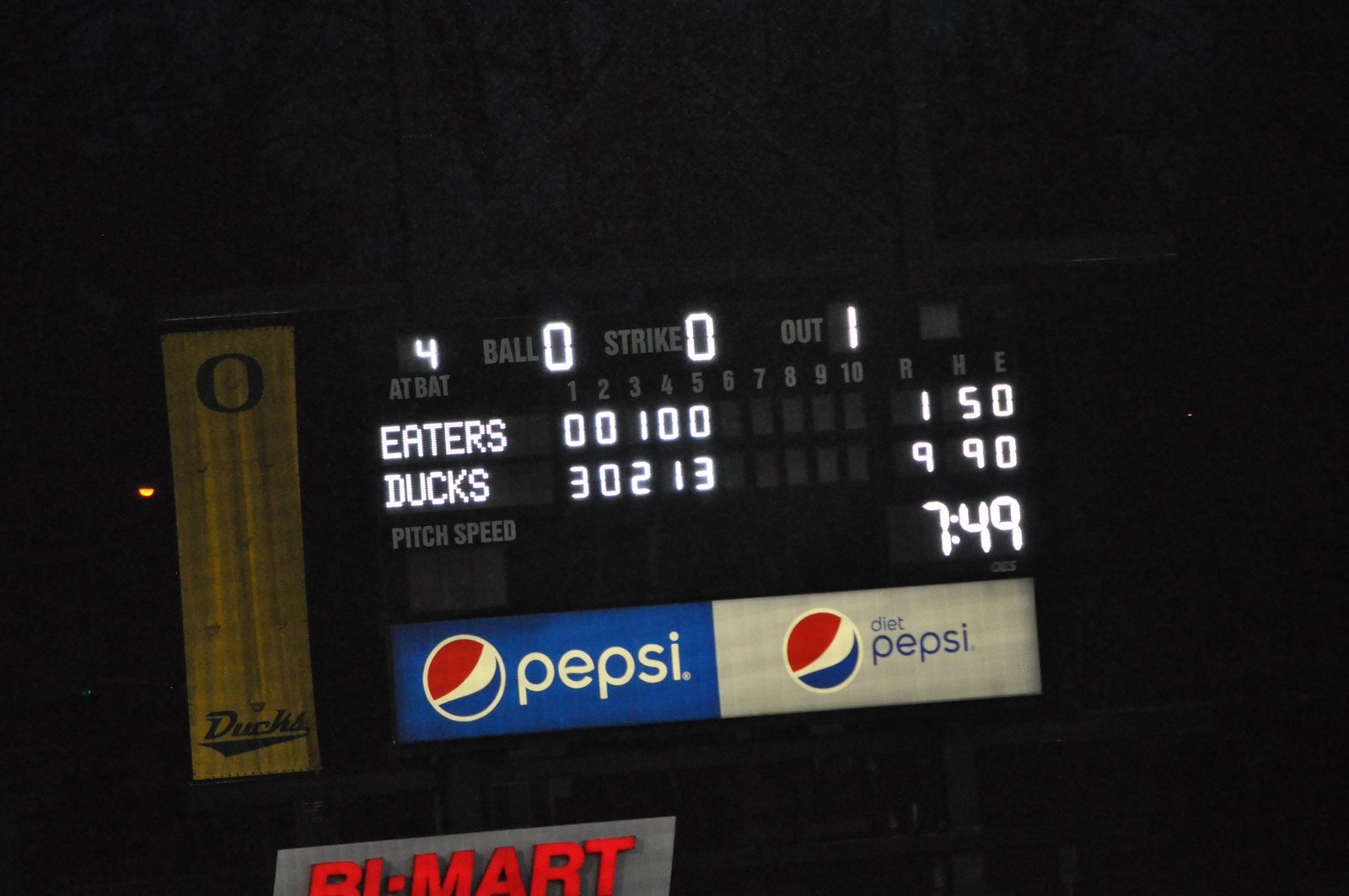This image captures a nighttime scene of a baseball scoreboard with a dark background, taken straight-on. The scoreboard is supported by visible metal beams. On the left side, there's a prominent yellow banner midway down, featuring a black "O" at the top and the word "DUCKS" in black lettering at the bottom, underlined by a thick black line. The scoreboard displays essential game information: a lit-up "4" under "AT-BAT", "BALL" with a lit-up "0", "STRIKE" with a lit-up "0", and "OUT" with a lit-up "1". The teams listed are the EATERS, with a score of 1 run and 5 hits, and the DUCKS, leading with 9 runs and 9 hits. Below the scores, the time reads 7:49 PM. At the bottom of the scoreboard are two rectangular Pepsi advertisements: one with a blue background and the Pepsi logo alongside white lettering, and another with a silver background, the Pepsi logo, and blue lettering for Diet Pepsi. Beneath the first Pepsi sign, a gray sign with red lettering reads "BUY MART."